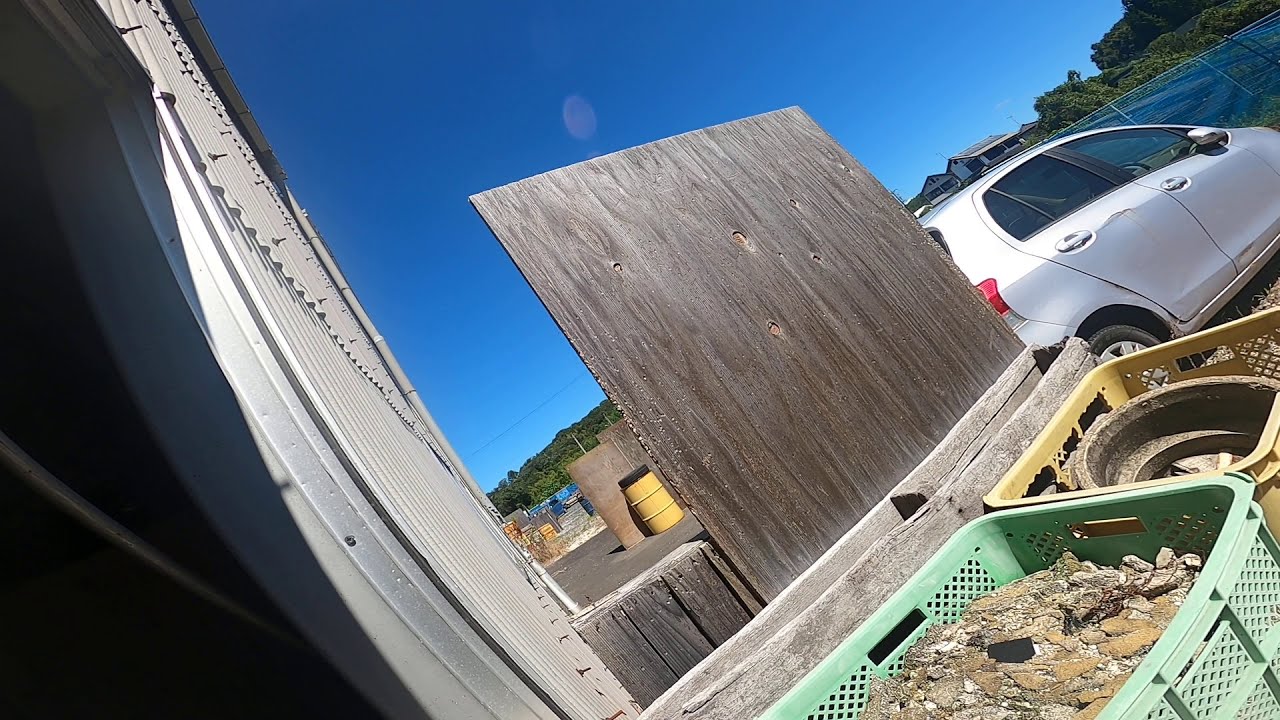This photograph captures an outdoor scene where various elements are juxtaposed against a white-painted building wall on the left. Prominently featured on the ground are two baskets: one green, filled with dirt, rocks, and sand; the other yellow, containing a rusted metal object, likely a vehicle rim. These baskets are placed beside a weathered piece of plywood standing upright, suggesting makeshift sorting of debris. A silver, four-door compact car is parked up against a blue-colored chain-link fence on the right side. Beyond the fence, other houses and trees can be seen, adding depth to the background. Further details include a yellow trash container on the left, a golden-colored barrel in the distance, and a clear, bright blue sky overhead. The composition and angle of the photograph create a detailed, multifaceted snapshot of an outdoor setting in a residential or semi-industrial area.